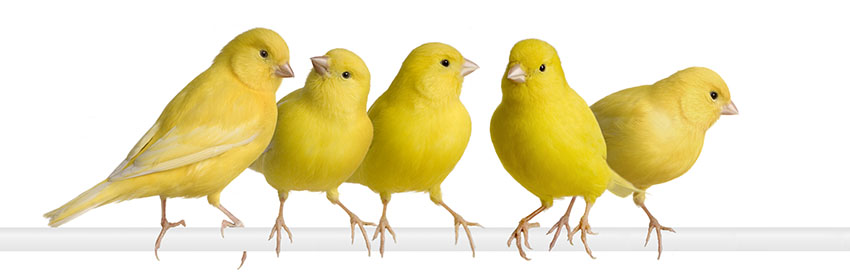In this captivating close-up photograph, five small, bright yellow birds are perched on a solid white bar that runs across the bottom of the image. The stark white background accentuates the vivid yellow of their feathers. These birds, with their stick-like legs and yellowish-orange claws, are positioned in various stances. The first bird, standing with its back to the camera, turns its head around, revealing black dot-like eyes and a pearly white beak. The second bird appears to be looking at the first, while the third bird faces directly to its left. The fourth bird stares straight ahead, seemingly engaged with the viewer, and the fifth bird, partially obscured by the fourth, looks sharply to its left as if ensuring no funny business. Their uniform appearance is detailed by their tucked wings and tails, black eyes, and light brown triangular beaks, enhancing the harmony and intrigue of their ensemble.